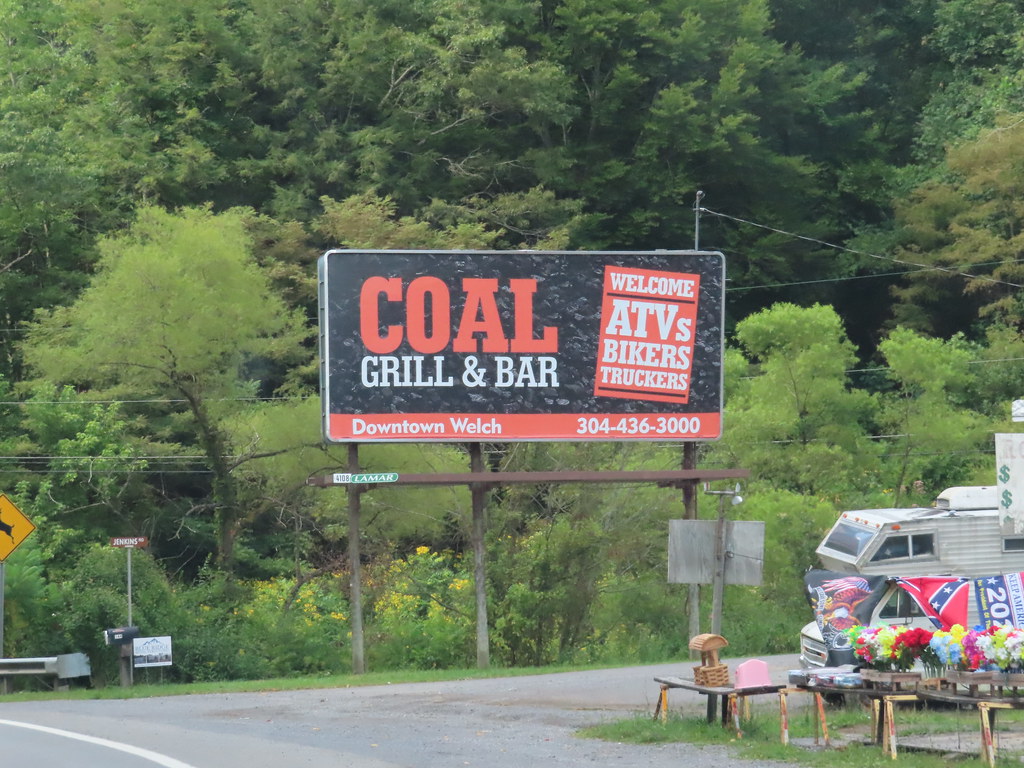In this outdoor scene, the focal point is a large billboard prominently situated on three wooden poles by the side of a paved road that veers off to the left, as indicated by a white line and a partially visible deer crossing sign. The billboard advertises the "Coal Grill and Bar" with bold, orangey text against a black background resembling actual coal, welcoming ATVs, bikers, and truckers. Below this on a red-bordered section, it lists "Downtown Welch" and a phone number, 304-436-3000. The area surrounding the billboard is densely wooded, with thick forest-like trees in the background. To the right of the billboard, there is an RV, several flags including a Confederate flag, and an array of flowers on tables, suggesting a market or roadside stop. Additional signs and a mailbox are visible below and to the left of the billboard, enhancing the roadside ambiance.